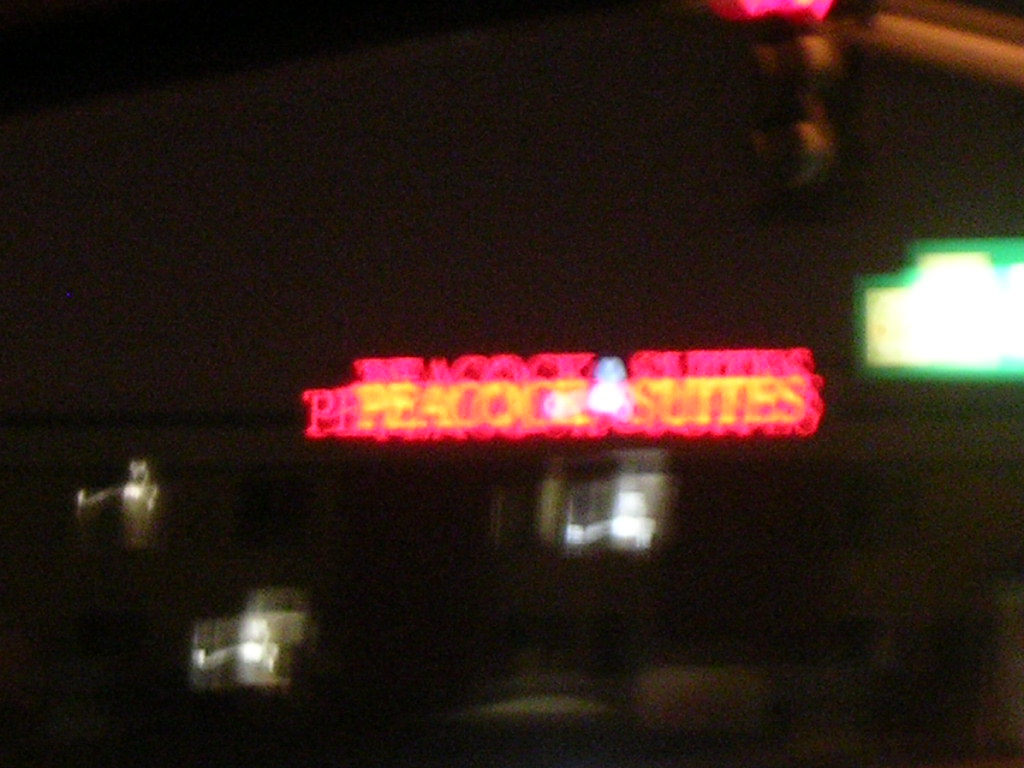A blurry nighttime photograph, seemingly captured from a moving car, depicts an illuminated urban scene. At the center of the photograph stands a building topped with a neon sign reading "Peacock Suites." Due to the motion blur, the sign appears multiplied and stretched, with the letters transitioning from orange to a stretched red hue. The building is two stories high, with three lights visible: one centrally located directly below the sign and two on the left side, one on each floor. To the top right of the image, a traffic light hangs down, with its red light glowing and also appearing blurred and duplicated. In the bottom right corner, a green road sign reflects car headlights, creating a bright white blur in the center. The sky is pitch black, adding contrast to the illuminated elements within the frame. Additionally, a light pole on the right side of the photo casts illumination on the traffic light pole, enhancing the nighttime atmosphere.